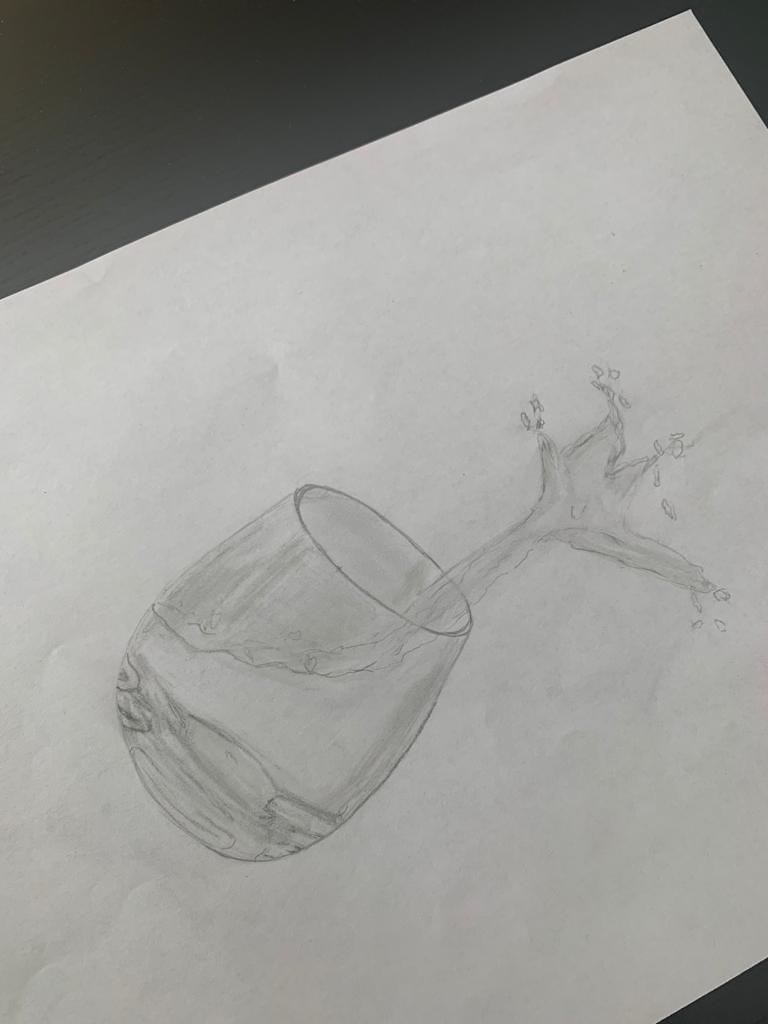This photograph captures a detailed drawing rendered on a piece of white paper, possibly sketchbook paper, newsprint, or printer paper. The drawing, executed in black and white, features a highball glass that appears tilted at an angle. This tilt causes the liquid inside to dramatically spill out, creating an explosive effect. The medium used seems to be pencil, sketch pencil, or charcoal, with visible shading and blended lines, particularly towards the top of the glass. Careful highlights and intricate details adorn the bottom of the glass, adding depth and realism to the artwork.